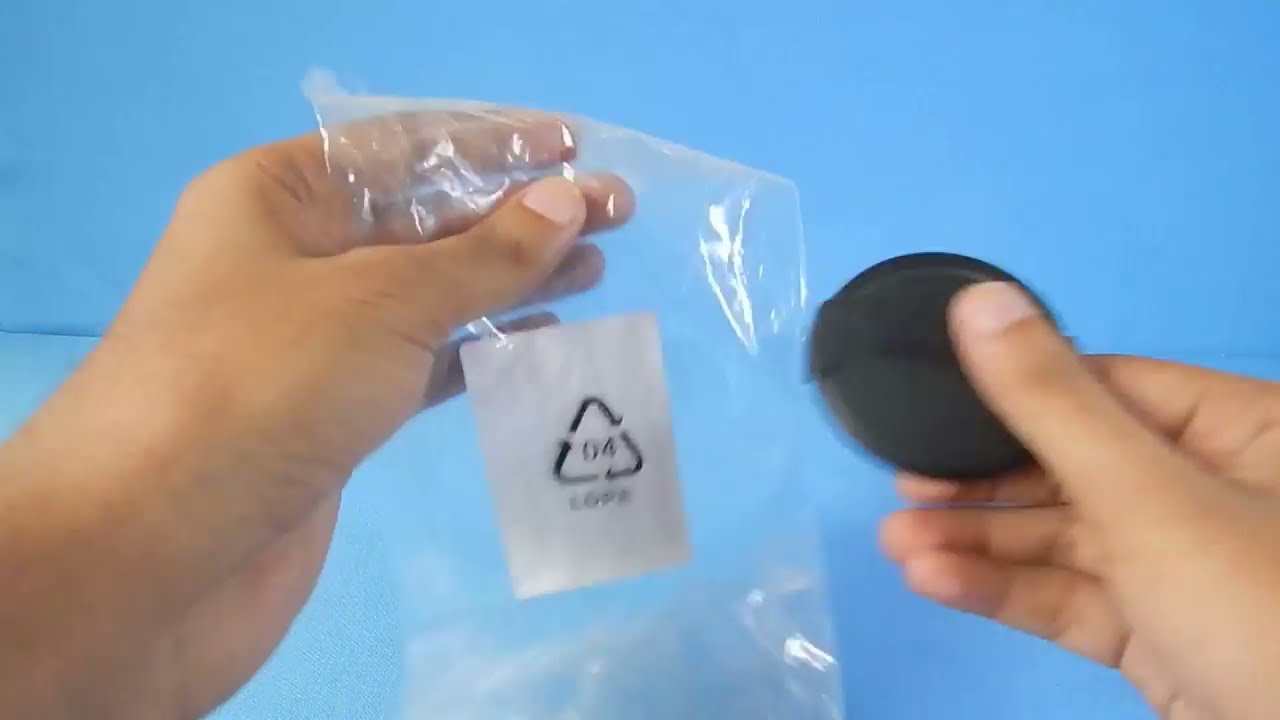The image features a person conducting an unboxing video of an electronics product. The setting includes a light blue backdrop, which highlights the silver and black components being showcased. Central to the image are a pair of hands meticulously untying a black cord, which features a standard USB connector on one end and a mini USB connector on the other. The hands are prominently positioned, with a twist tie being removed from the cord. In the background, various pieces of electronics are visible, including what appears to be a Samsung device and several black cases. Additionally, a cylindrical object can be seen near the right hand. The contrast between the black cord and the silver ends, along with the array of neatly arranged electronic items, creates a clear focal point for understanding the unboxing process.